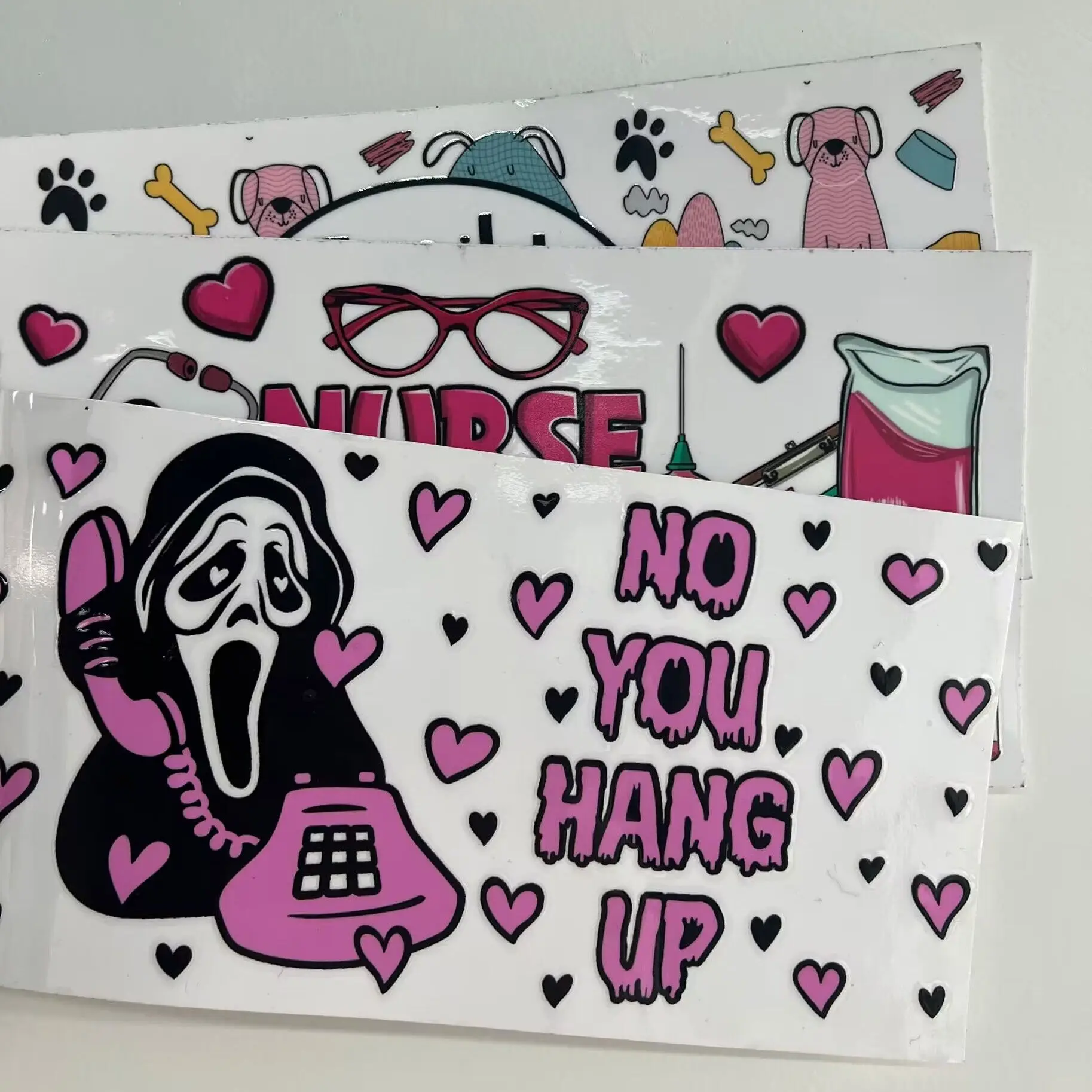The image displays three overlapping, rectangular posters with various designs. The foremost poster has a white background adorned with purple and black hearts. Prominently featured on the right side, large purple letters outlined in black spell out "KNOW YOU HANG UP," each word stacked vertically. The letters have a dripping effect, mimicking wet paint. To the left, a graphic of the Scream movie's ghost mask in a black hood and robes appears, holding a retro purple phone with a coiled cord and square buttons. Notably, the mask has hearts in its eye sockets.

The middle poster is partially visible and showcases a pair of red glasses at the top. Scattered around are red hearts, and the readable part of the text says "NURSE" in pink. A syringe and stethoscope in red and blue hues are faintly visible on the right side.

The third, most obscured poster features a whimsical, dog-themed design. It includes a collection of small, colorful illustrations: a black paw print, yellow dog bones, pink and blue dogs with floppy ears, and a blue dog dish.

The posters collectively create a collage of playful and contrasting elements, merging horror and cuteness.